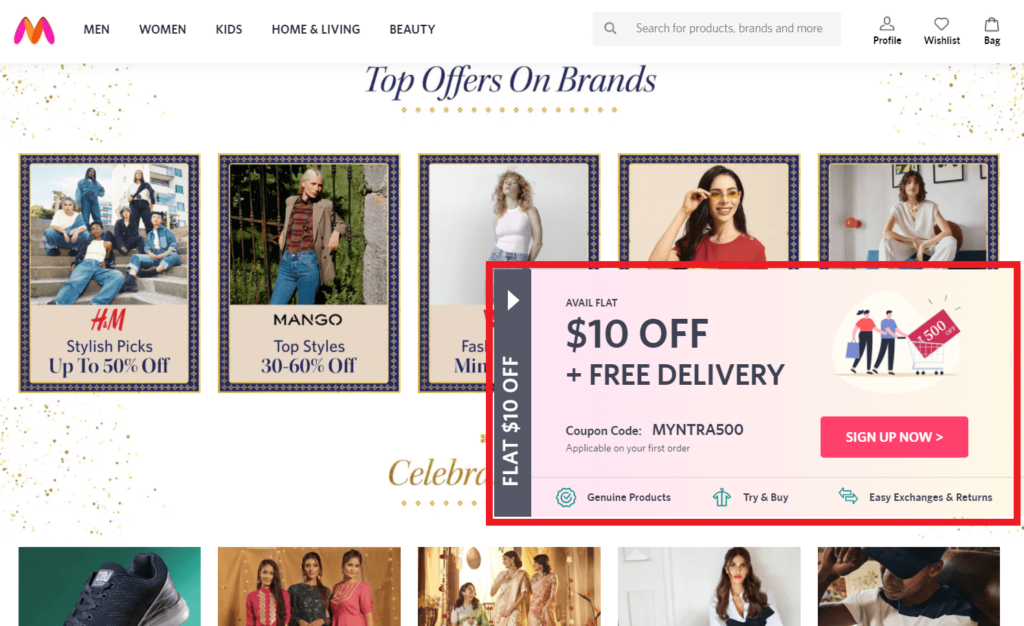This image is a cropped screenshot depicting a portion of the home page of Myntra, an Indian e-commerce company specializing in fashion and lifestyle products. At the top left corner, the Myntra logo, an 'M' in shades of pink and red, is prominently displayed. To the right of the logo, various shopping categories such as Men, Women, Kids, Home & Living, and Beauty are listed horizontally across the header. Next to these categories, a white search box features the placeholder text "Search for products, brands, and more" in small gray letters. Further to the right, icons for profile, wishlist, and shopping bag are aligned.

The main body of the website features a clean white background adorned with small confetti decorations on the left and right margins. At the top center, a bold black headline reads "Top Offers on Brands," emphasized by a horizontal line of gold stars beneath it.

The page's central area is organized into a grid layout of square photo thumbnails, each showcasing models in various fashionable outfits. Superimposed on the center-right part of the page is a prominent $10 off plus free delivery coupon, which is encased in a red outline. The text "$10 off plus free delivery" is presented in large letters. Below this offer, on the left, the bold black text "Coupon Code" is displayed alongside the specific coupon code. Towards the bottom right of this overlay, a red "Sign Up Now" button invites users to take advantage of the offer.